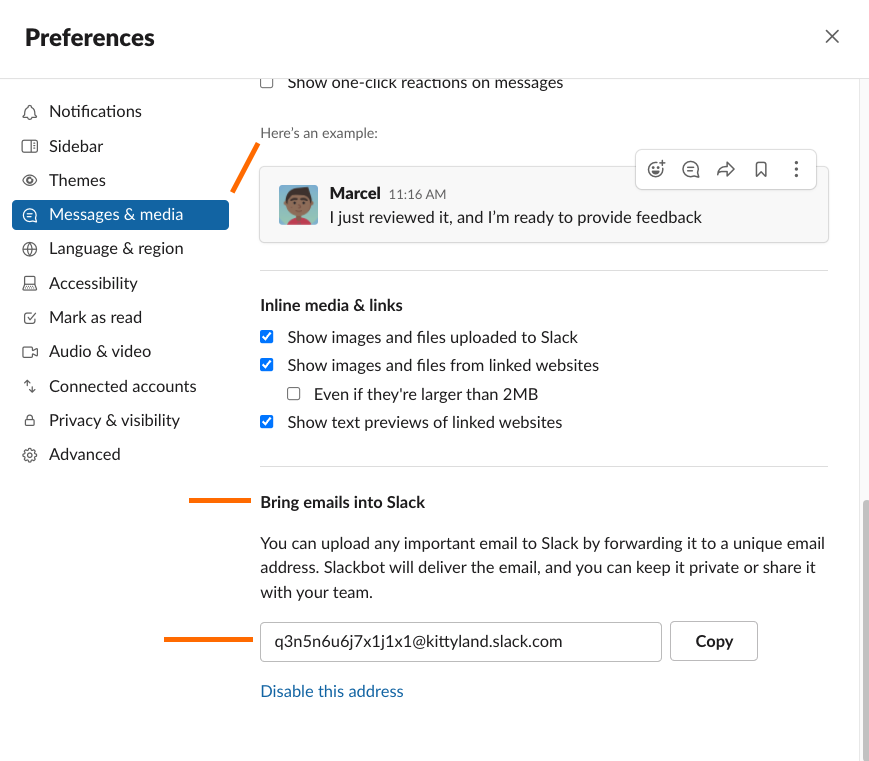**Detailed Caption:**

The image is a screenshot of the "Preferences" section in a software application interface, prominently labeled in bold black letters at the upper left corner. A vertical sidebar on the left lists various preference options, where "Notifications," "Sidebar," "Themes," and "Messages and Media" are clearly highlighted, indicating the currently selected option. Other available but unselected options include "Language and Region," "Accessibility," "Mark as Read," "Audio and Video," "Connected Accounts," "Privacy and Visibility," and "Advanced."

The focus is on the "Messages and Media" subsection. The topmost setting in this section displays the option "Show one-click reaction to messages," followed by an illustrative red line annotated with "Here's an example." The example is a replicated message from "Marcel" (timestamped at 11:16 AM) with the text stating, "I just reviewed it, and I'm ready to provide feedback."

Below this example, there is a series of settings related to media and inline links:
- A checked box next to "Show images and files uploaded to Slack."
- Another checked box for "Show images and files from linked websites."
- An unchecked box for the option "Even if they're larger than 2 megabytes (MB)."
- A subsequent checked box for "Show text previews of linked websites."

Further, an orange horizontal bar labeled "Bring emails into Slack" explains the functionality of forwarding important emails to Slack via a unique email address. This is followed by a description that Slackbot will deliver the emails, which can then be kept private or shared with the team.

Lastly, below another orange vertical bar, there is an input field containing a long, seemingly random email address: "Q3N5N6U6J7X1J1X1@kittyland.slack.com." To the right of this email address, there is a "Copy" button for easy copying, and a blue selectable field labeled "Disable this address" is also present.